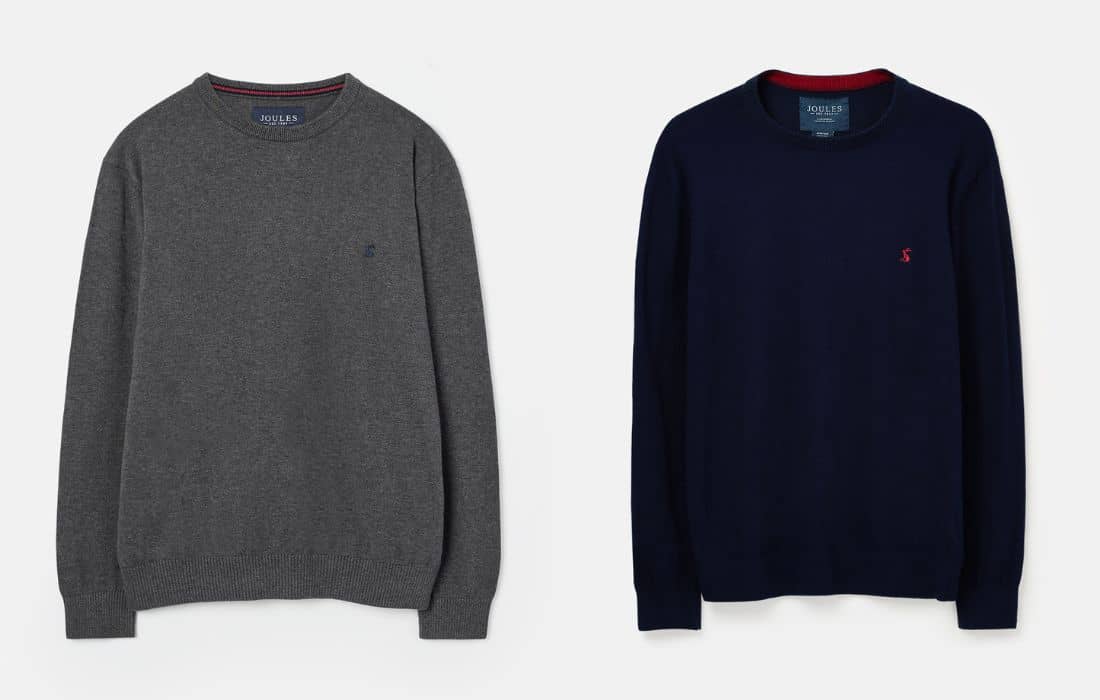The image shows two long-sleeved sweaters displayed on a pale background. Both sweaters feature a round neck with trimming and belong to the designer brand Jules, indicated by a label inside the neck of each sweater. The sweater on the left is grey, while the one on the right is navy blue (black in certain lighting). Both garments display a logo on the front chest, although its detail isn't fully clear. The inside collar of the grey sweater has a thin orange line, while the navy blue sweater features a red line along the back of the collar. The collars appear slightly different, with the navy blue sweater's collar being slightly lower in the front. These sweaters are likely designed for men, based on their style and fit.